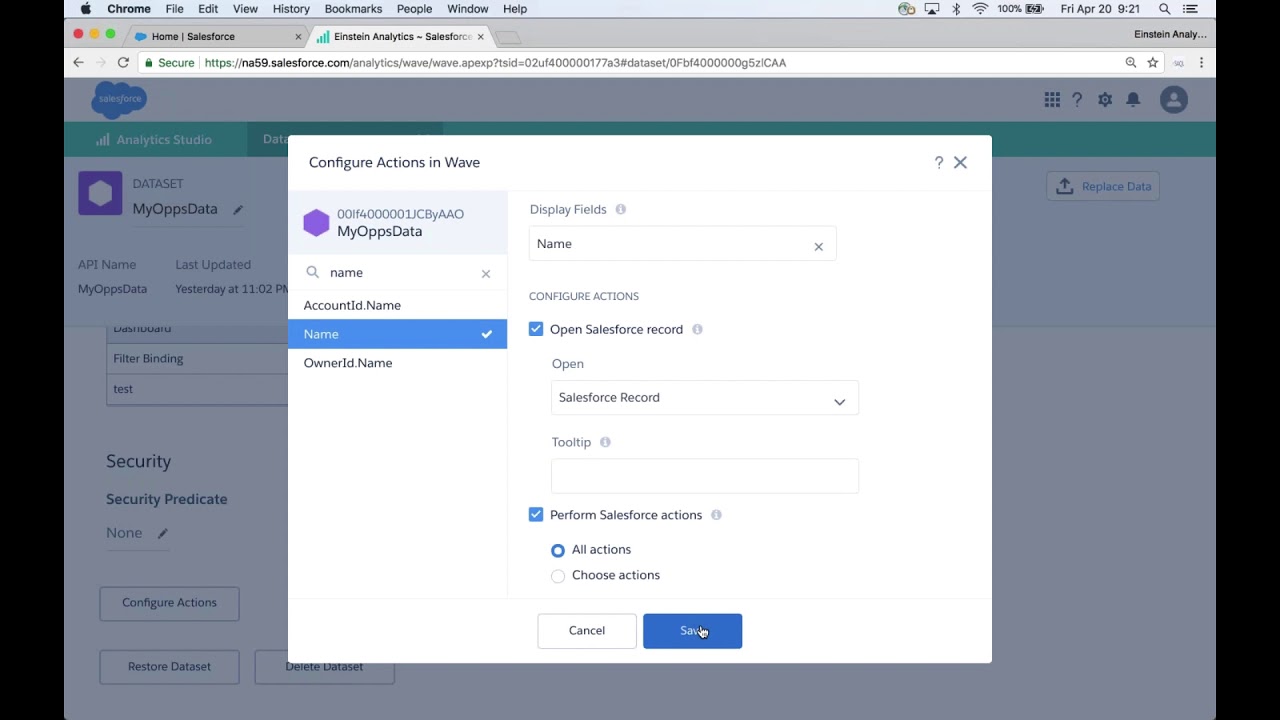This image appears to be a screenshot taken from a computer screen, capturing an interface of a software application. The edges on both the left and right sides of the screen are fully black, forming almost rectangular borders. The central part of the screen displays a light blue rectangle containing various pieces of information. Positioned prominently on top of this section is a white rectangular box with detailed text.

At the top of the white box, in bold black print, the text reads "Configure Actions in WAVE." Beneath this header, the interface references data titled "My Ops Data," accompanied by a long numerical string. Adjacent to this string is a purple hexagon icon.

This interface includes several labeled fields - "Name," "Account ID Name," "Owner ID Name," and more. There are also display fields marked "Name" and "Configure Actions." Within these sections, the user has selected "Open Salesforce Record." 

Further down, under the header "Perform Salesforce Actions," there are options for "All Actions" or "Choose Actions," with the "All Actions" option highlighted in a light shade of blue. At the bottom of the white box, two buttons labeled "Cancel" and "Save" are visible. Of note, the user's mouse, represented by a hand icon, is hovering over the "Save" button, indicating the user's intent to save the configurations.